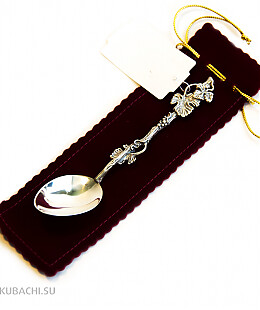This image is a detailed capture of a collectible miniature spoon, typically treasured by collectors who display them in specialized cabinets. The spoon is elegantly laid on top of its carrying pouch, which is crafted from a luxurious black velvet material. This pouch is distinctively finished with a crimped edging and is secured by a gold drawstring at the top.

The spoon itself is metallic, appearing somewhere between gold and silver, possibly due to the lighting. It features an intricately ornate handle adorned with a floral and vine design. There's a small white tag attached to the spoon, though any writing on it is indiscernible.

Beneath the spoon, in the bottom left corner of the pouch, are the letters K-U-B-A-C-H-I-dot-S-U, adding an additional layer of authenticity and origin to this collectible item.